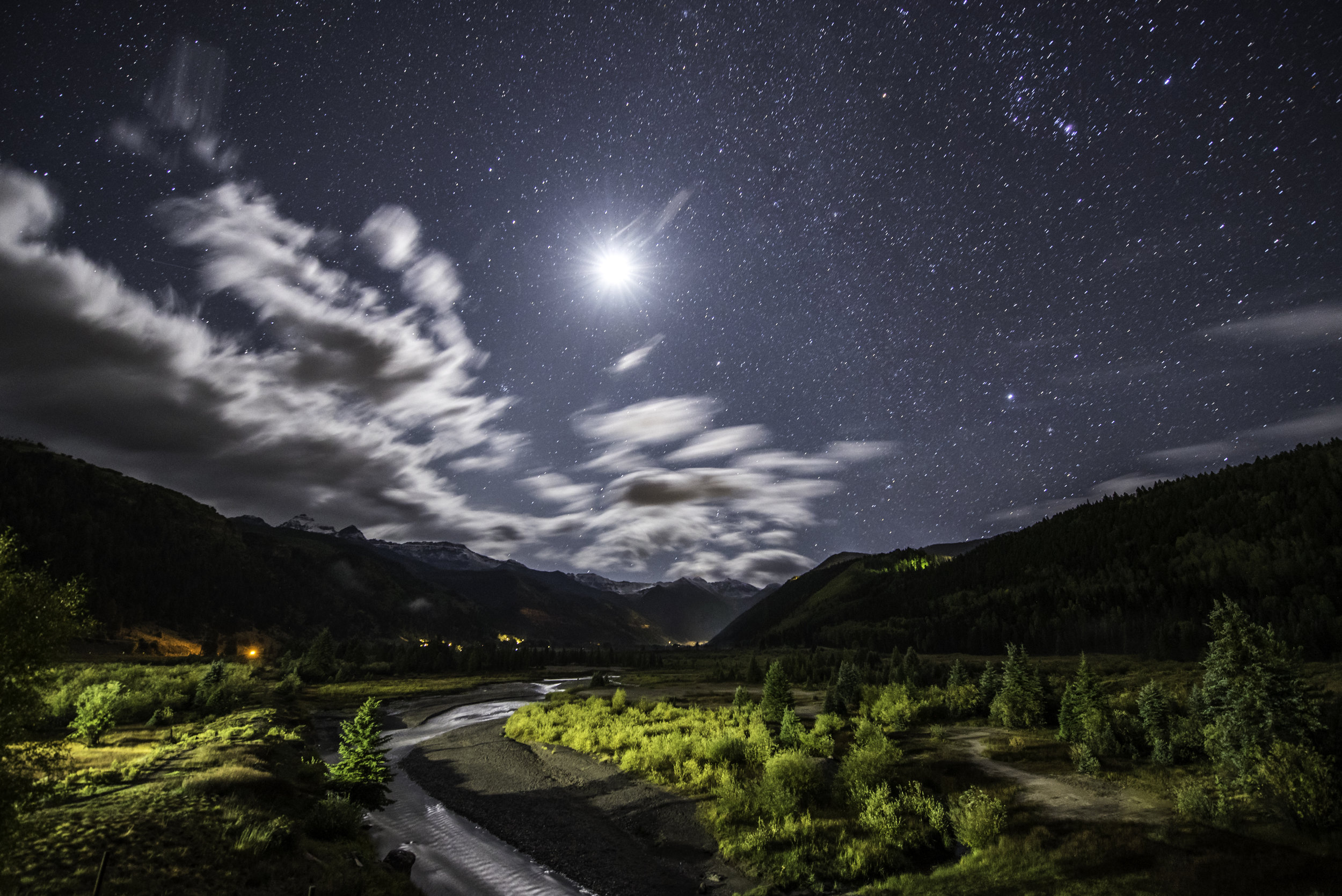This nighttime landscape photograph features a breathtaking scene with various natural elements meticulously detailed. The expansive night sky is a deep blue, dotted with numerous stars, and dominated by a singular, exceptionally bright star that radiates prominently at the top center. To the left, dynamic, white fluffy clouds appear blurred, suggesting movement against the backdrop of the sky. Below, a serene river winds through the middle of the landscape, flanked by verdant green trees and foliage. The river is bordered by dark, clean, and imposing mountain ranges that converge towards the center, with inclines descending from the left and ascending towards the right, creating a harmonious middle convergence. At ground level, a winding road curves gently from the bottom middle of the image to the left before veering back to the right. Scattered lights glow warmly from houses nestled on either side of the mountains, adding a touch of human presence to this otherwise pristine, starry night scene.